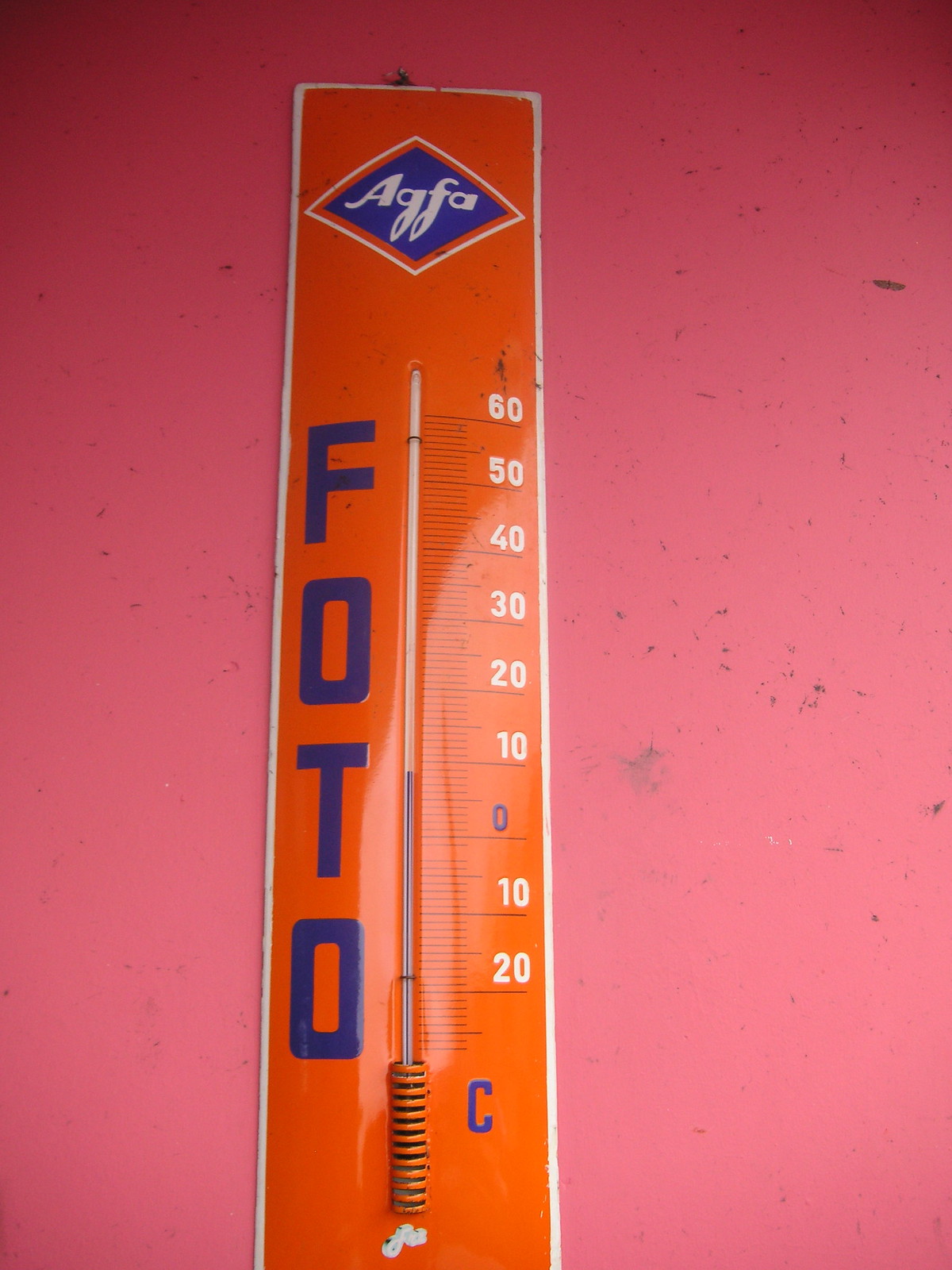This photo showcases a vintage temperature gauge, designed with a sleek and elongated profile, crafted entirely out of metal. The thermometer, painted a vibrant orange, is mounted on a wall, adding a pop of color and a touch of retro flair.

The top of the thermometer features a distinctive diamond shape, proudly displaying the brand name 'AGFA' in bold white letters against a blue background. The central part of the gauge consists of a mercury-filled tube, which accurately measures the ambient temperature.

On the left side of the temperature gauge, the term 'FOTO' is inscribed in dark blue letters, indicating its photographic application roots. On the right, a series of numerical markers gradually descends from 60 at the top to zero, with additional lines extending down to 20. At the bottom of the scale, a prominent 'C' signifies that the readings are in degrees Celsius.

The current reading on the thermometer is approximately 9 degrees Celsius. A small cylindrical piece is positioned beneath the mercury tube, serving as its reservoir and enhancing the overall vintage aesthetic of this functional and stylish temperature gauge.